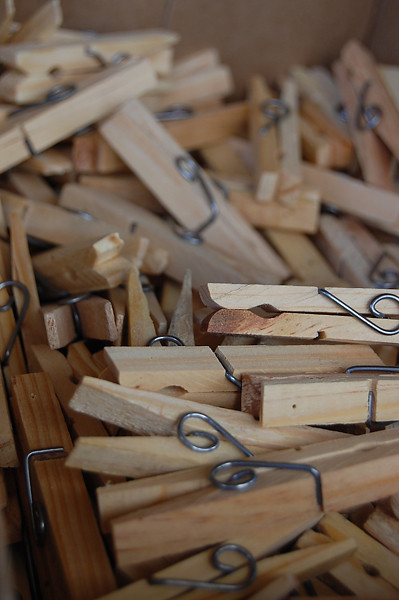This vertically oriented color photograph captures a vibrant scene of over 60 wooden clothespins piled haphazardly in an abstract arrangement. The clothespins, made from light-colored wood with visible tree grain markings, feature a sleek silver wire clip in their center that facilitates opening and closing. The image is brightly lit, suggesting it was taken in a well-lit room, though there is a shadowy area in the left-hand corner. The central clothespins are in sharp focus, with those at the top and bottom appearing blurred, adding depth to the composition. Notably, one clothespin in the center has a darker brown shade near its tip. The overall tint of the photograph is a reddish sepia, enhancing its artistic quality.